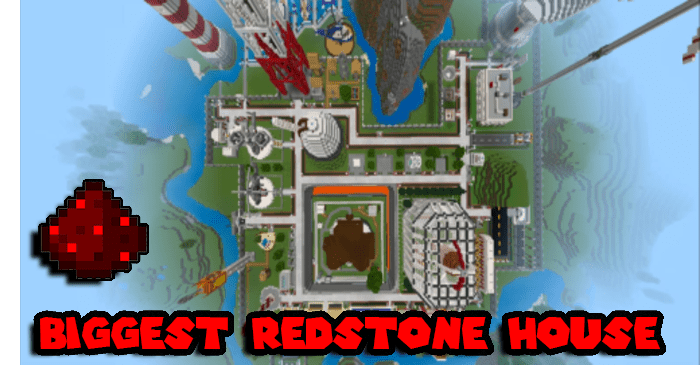This image is an overhead, rectangular view of a digitally animated game, likely from an older computer or video game like Minecraft. The scene is characterized by a vibrant, cartoonish landscape featuring Lego-like buildings and structures. At the bottom of the image, bold red text with a black outline prominently reads "Biggest Redstone House." The terrain suggests water boundaries resembling either an ocean or lake surrounding the city, with noticeable water scenery on the far left and right, slightly faded as if seen through clouds.

The upper left section showcases a tall, red-and-white striped lighthouse, extending beyond the visible frame. Centered within the scene, clear white and gray lines—resembling roads or pipes—crisscross horizontally and vertically, indicating complex connection points. These lines intersect amidst various buildings, many appearing white and clustered towards the top of the image. In the upper right, a tall silver pole with a flag is partially visible, extending out of frame.

Below the text, there's a conically shaped structure, pixelated and brown with six bright red squares on top, adding to the game's stylized aesthetic. Grassy areas intersperse the buildings, contributing to the lush, green expanses within the city grid, while the brown-and-red dotted island in the left portion of the image further showcases the pixelated, blocky artistry typical of older video games.